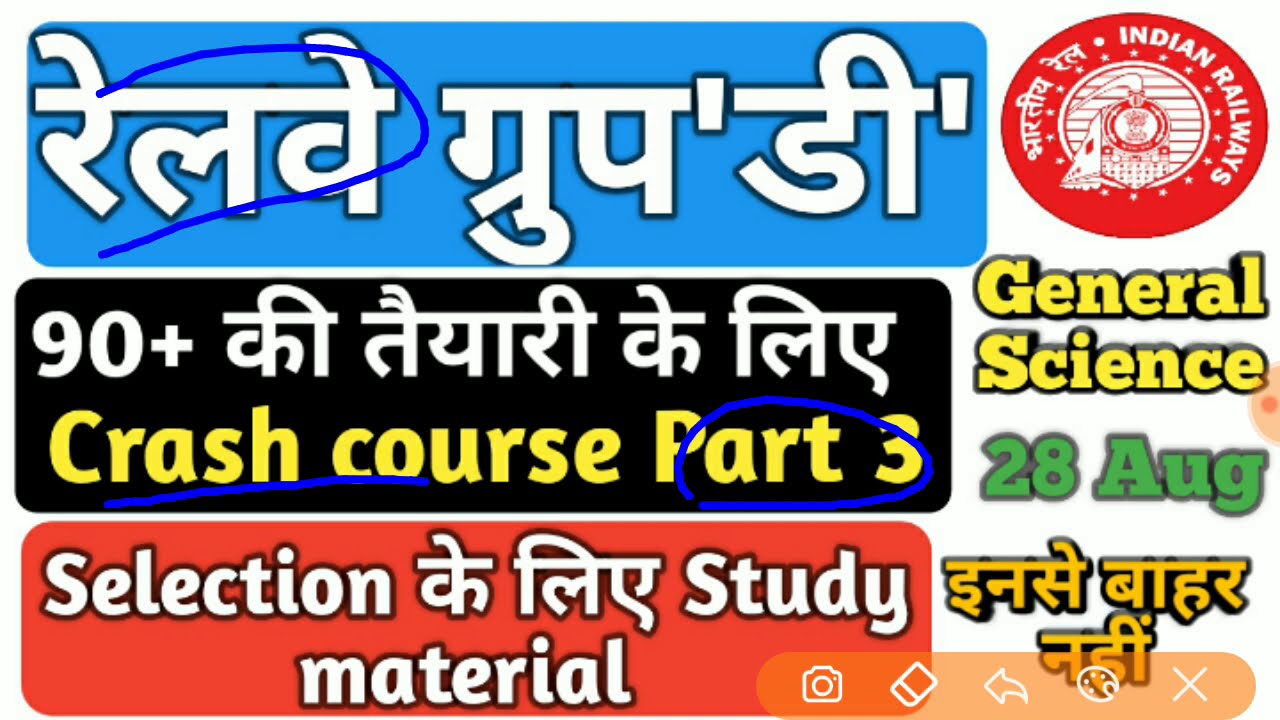This image appears to be a high-definition slide or poster promoting a seminar or course for Indian Railways. The design is segmented, with three long, horizontal sections on the left side, each in different colors—blue at the top, black in the middle, and orange at the bottom. These segments contain white text, written predominantly in what seems to be an Indian script. 

The middle section features additional text in English with "Crash Course Part 3" written prominently in yellow, where "Part 3" is circled in blue, and "Crash Course" is underlined in blue. Below this, the orange section reads "Selection Study Material" in white text, following a similar layout of English and Indian script.

At the top right, there's a circular orange logo with a white center and an illustration of a train. Surrounding this logo, it reads "Indian Railways" in white text. Directly below the logo, the text "General Science" is displayed in yellow, followed by "28th August" in green. Additional symbols and icons, including a camera and various action symbols, are found beneath this.

The overall impression is that of an informational and promotional piece for an upcoming event or course, possibly a seminar or training session, related to Indian Railways, focused on General Science. The various colors—blue, black, yellow, red, white, green, and orange—add to the visual segmentation and emphasis.